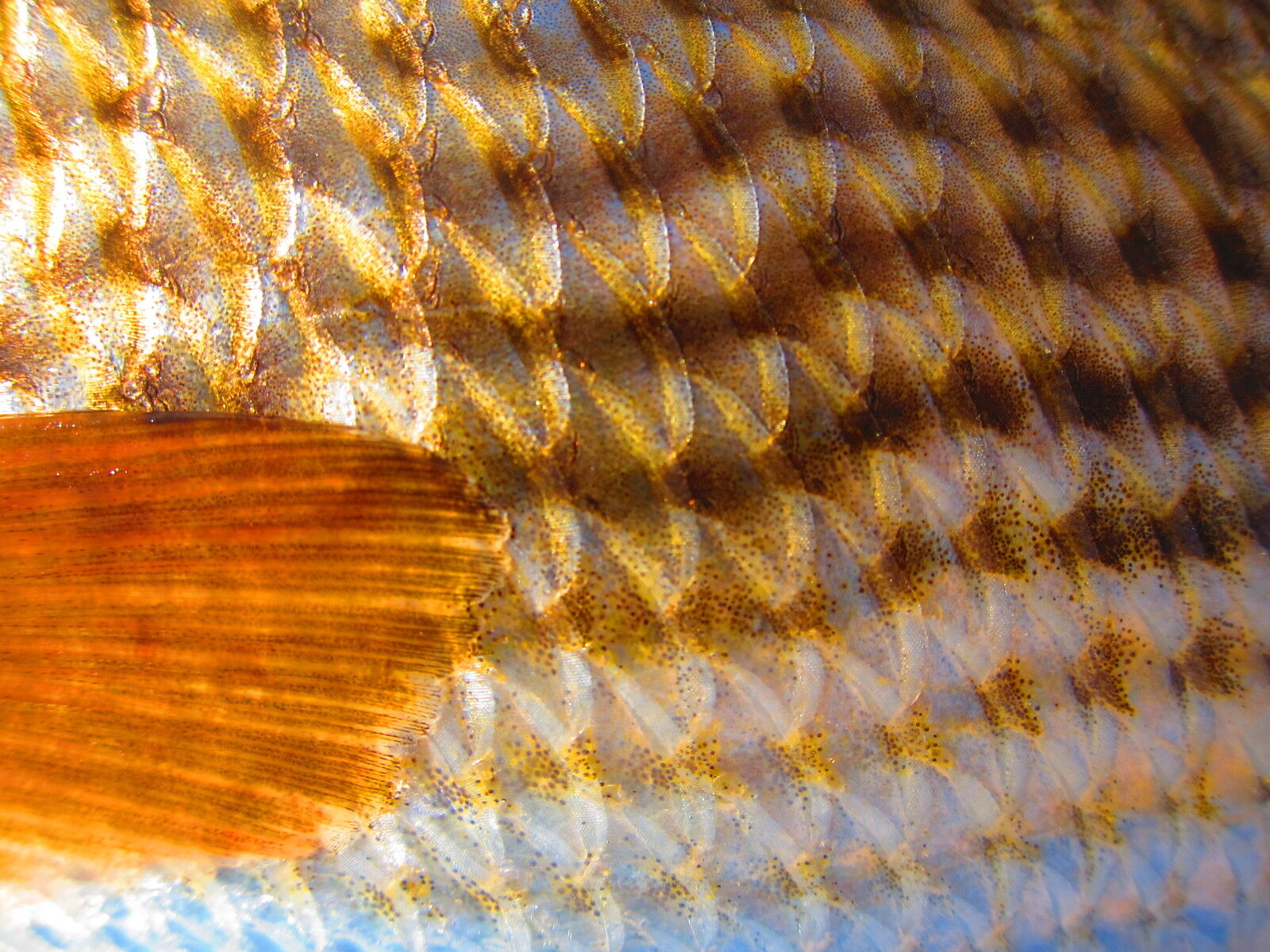This extremely close-up photograph captures the intricate details of a goldfish's scales and fin, filling the entire frame. Dominated by rows of U-shaped scales, the colors alternate between dark brown, yellow, and shimmering gold, with intermittent splashes of orange hues. The upper portions of the scales exhibit a complex pattern of dark brown that gradually transitions into lighter tones towards the bottom, where shades of gold, yellow, and white become more prominent. In the bottom left corner, a fin is noticeable, its color transitioning from a burnt brown-orange at the top to a lighter yellow at the bottom. The fin extends along the goldfish's side, occupying nearly half of the image vertically and a portion of the left-hand side horizontally. The lighting in the photograph is bright, enhancing the clarity and vividness of the fish's detailed textures.